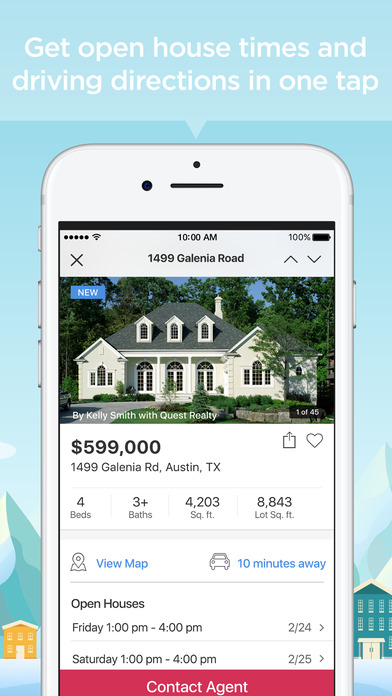The advertisement showcases a convenient feature for finding open house times and driving directions with a single tap. Set against a light blue background, the image features a row of charming houses near the bottom. On the left, there's a small orange house, while a blue house stands on the right. The backdrop includes fluffy clouds and distant mountains adding to the scenic beauty. At the center of the image, there's a depiction of an iPhone screen displaying detailed information about a specific property.

The iPhone, showing 10 a.m. with a full battery, features data about a house located at 1499 Galenia Road. This home has a gray roof and white walls, with several windows enhancing its facade. The listing is presented by Kelly Smith from Quest Realty, with a price tag of $599,000. Key property details include four bedrooms, three bathrooms, a total living space of 4,203 square feet, and a lot size of 8,843 square feet. Additionally, the screen offers options to view the house on a map, with an indication that it is 10 minutes away, marked by a location icon and a car icon.